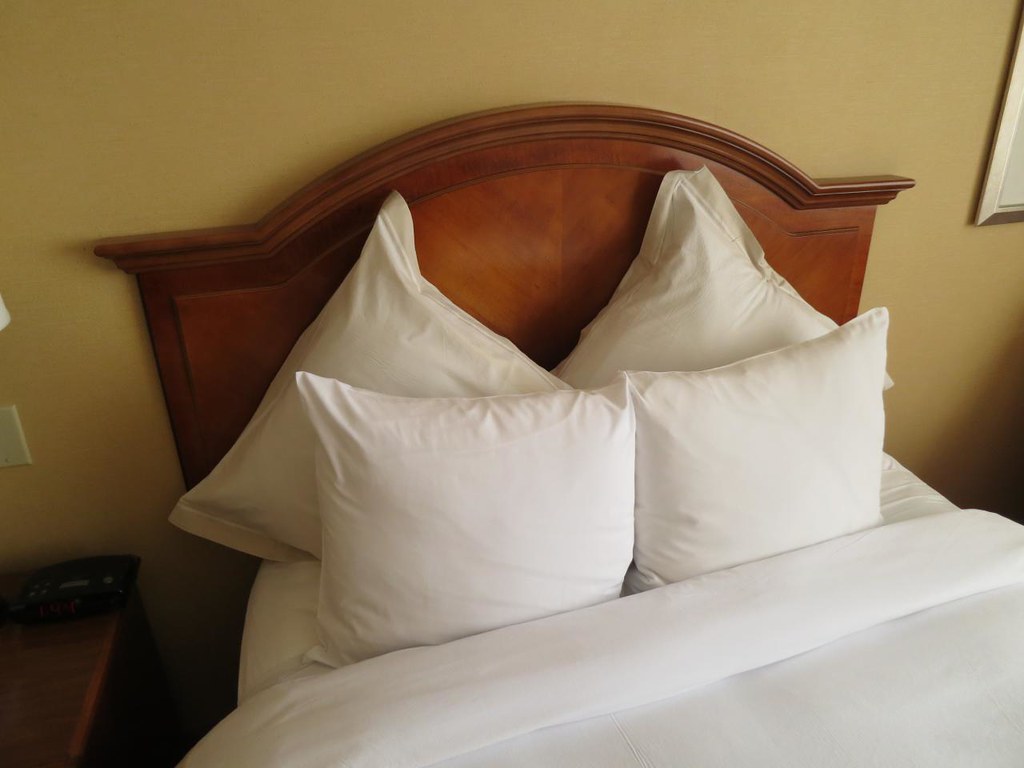This indoor color photograph depicts a well-made bed situated against a wall that appears to be a light yellow-green. The bed features pure white sheets and four matching white pillows. The wooden headboard, crafted from a rich mahogany with a subtle arch in the middle, adds an elegant touch and is placed directly against the wall. The arrangement of the pillows creates a visually pleasing composition: the two back pillows are square-shaped and angled so their points face upwards, while the two front pillows are rectangular, positioned on their longer edges. To the right of the bed, a partial view of a silver picture frame is visible in the upper-right corner of the image. Additionally, a dark brown wooden nightstand can be seen at the side of the bed, adding to the room’s warm aesthetic. The photograph captures a serene and meticulously arranged sleeping area without any text or additional decorations in the frame.